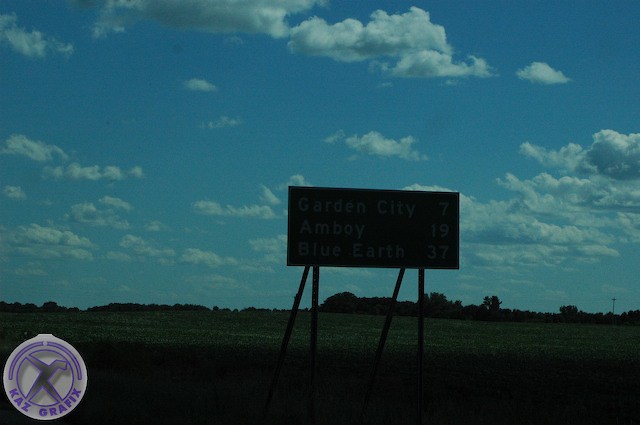The image showcases an expansive field, with the majority of the foreground cloaked in shadow. Standing prominently in this shaded area is a large hoarding notice elevated on long legs. Although the text on the hoarding is indiscernible, it stands out starkly against a vibrant blue sky adorned with clusters of white, fluffy clouds. A shadow, the source of which is unclear, partially darkens the hoarding and this section of the field. In the background, an array of trees and bushes adds a touch of greenery to the landscape. In the bottom left corner of the image, a white circular badge is visible, featuring the text "CATS graphics" in purple, along with an indistinct symbol.